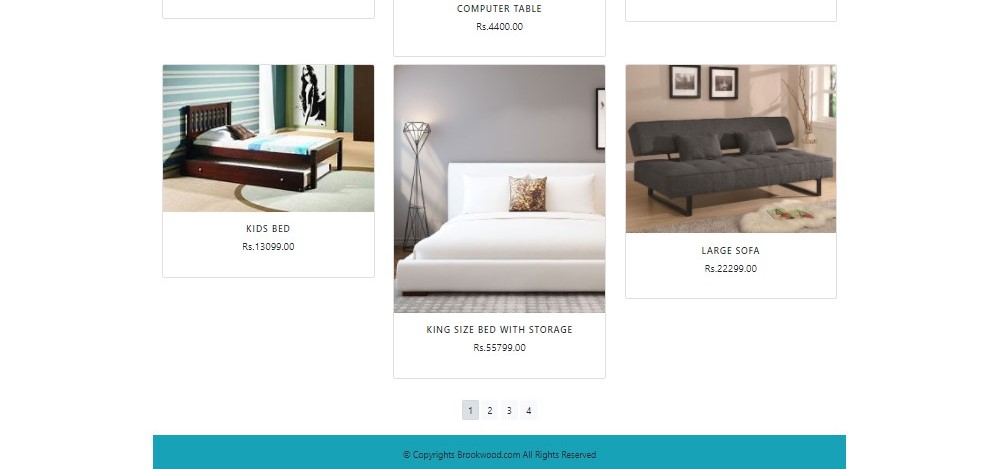This screenshot displays a section of a website showcasing a product gallery featuring various types of beds. The gallery is organized into three columns, each containing a distinct product. The first column highlights a kid's bed priced at RS 13,099. The second column showcases a king-size bed with storage, priced at RS 55,799. The third column features a large sofa that appears to be a fold-out, priced at RS 22,299. Each product is accompanied by a corresponding label and price mentioned in RS. Below the product images and prices, pagination controls are visible, indicating four pages in total through numbered buttons. At the very bottom, there is a two-colored bar indicating a copyright notice: "brookwood.com, all rights reserved."